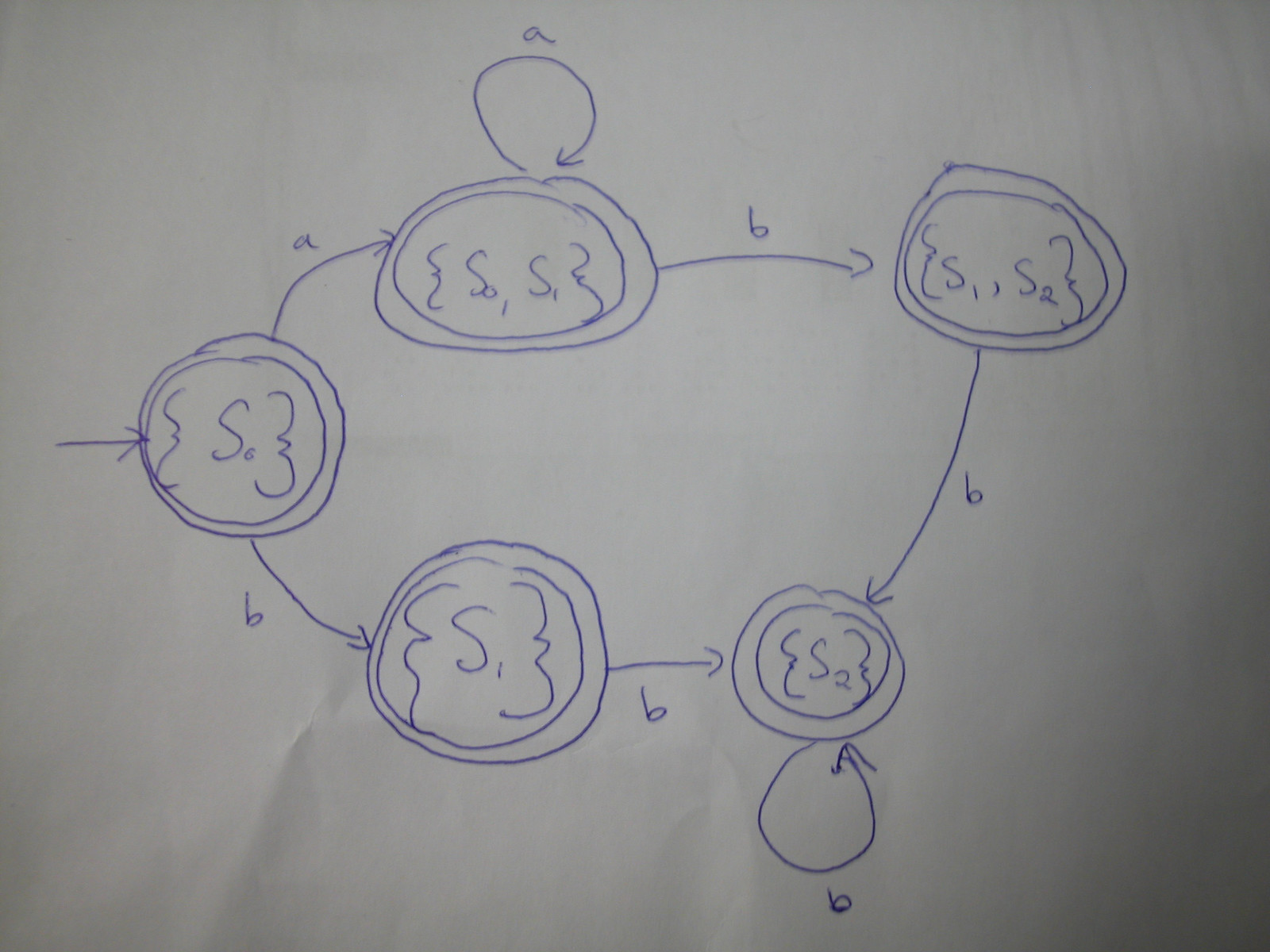A hand-drawn diagram on a slightly wrinkled piece of white computer paper. The entire diagram is rendered in blue pen ink. At the center of the composition are several circles, each encasing what appears to be text or symbols that resemble "C," "S0," and "S1," potentially indicating states in a state machine or placeholders for unspecified variables. Connecting these circles are arrows, also drawn in blue ink, which form a circular pattern around the central elements. The arrows are annotated with letters, primarily "A" and "B." Despite the organized layout, the exact purpose of this diagram remains unclear, leaving it ambiguous whether it represents a concept from mathematics, science, or another field.